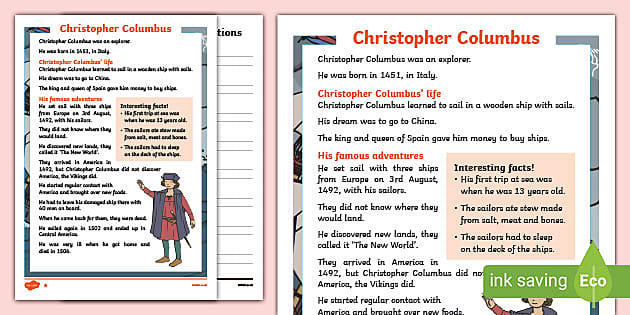This is an information card about Christopher Columbus, designed as an educational tool for young students. The card features a hand-drawn illustration of Columbus, printed on a pink background. He is depicted standing and waving, dressed in a red robe, a purple vest, green leggings, and light brown shoes. The top of the card reads "Christopher Columbus" in red text, followed by a brief biography in black text. It states that Columbus was born in 1451 in Italy and had a dream of sailing to China. Supported by the King and Queen of Spain, he embarked on his famous voyages. 

The card highlights key sections with red subheadings such as "Christopher Columbus's Life" and "His Famous Adventures." He learned to sail on wooden ships and set sail from Europe with three ships on August 3, 1492. Columbus’s voyages led to the discovery of new lands, referred to as the New World, although he did not recognize it as America. There's mention of regular contact with America and the introduction of new foods, although part of this text is obscured by an ink-saving eco symbol featuring a green leaf. 

The main card, printed on white paper with grayscale border accents, also features a small orange symbol in the lower left corner. Additionally, the design suggests it includes supplementary material, perhaps questions for students, to enhance learning. The text throughout the card is notably small, making it somewhat difficult to read.